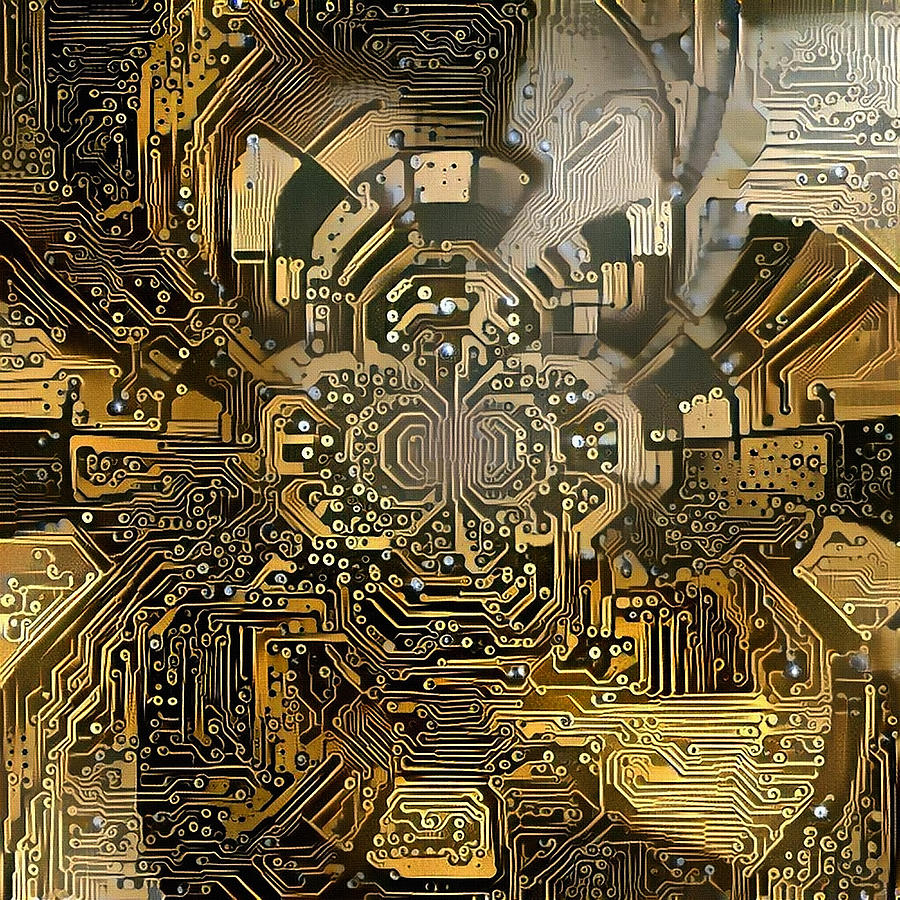The image depicts a detailed, artificially generated representation of a microchip or electronic circuit, heavily resembling a printed circuit board (PCB). The design is intricate, showcasing a complex network of digital connections, tiny screws, and conduits. The color palette is predominantly golden and brown, with interspersed blacks and light yellows, giving the board a metallic appearance. Central to the design is a spiraling pattern that adds to its intricate nature. The upper right portion of the image features a blurry brown-greyish shade, possibly indicating light. The style is akin to digital art with a futuristic, advanced technology theme, and no visible borders or text. The overall layout bears a striking resemblance to a computer motherboard, with its busy, detailed patterning and the square outline adding to the visual complexity.